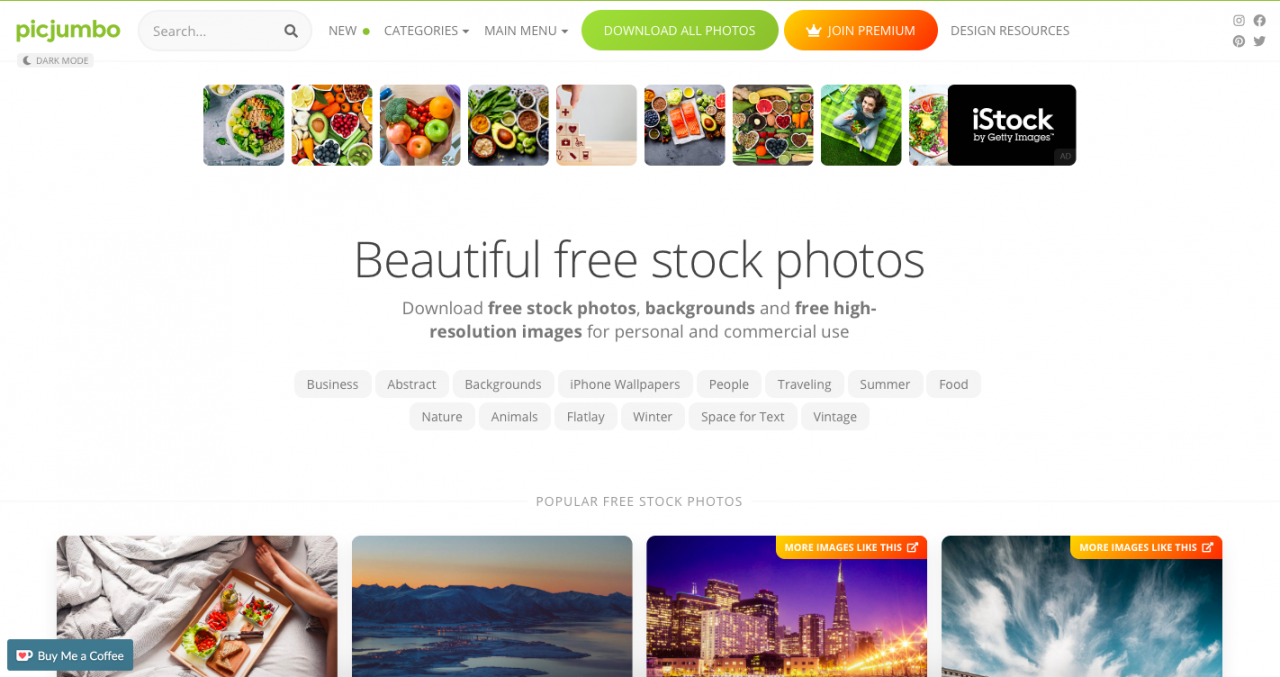The landscape-oriented image predominantly features a white background with the upper left corner displaying the logo "PIC Jumbo." Adjacent to this logo is a search bar, followed by options labeled "New," "Categories," and "Main Menu." To the right, a green button prompts viewers to "Download All Photos," while an orange button encourages them to "Join Premium." Additionally, a section for "Design Resources" is visible.

Central to the image are various stock photos including vibrant vegetable dishes, colorful salads, fresh fruits, and a woman lounging on a green blanket. On the right side of the image, the watermark "iStock by Getty Images" is discernible. Below, text advertises "Beautiful free stock photos," "Download free stock photos," "Backgrounds," and "Free high-resolution images for personal commercial use." 

A series of categorized buttons follows, offering options such as "Business," "Abstract," "Backgrounds," "iPhone Wallpapers," "People," "Traveling," "Summer," "Food," "Nature," "Animals," "Flat Lay," "Winter," "Space for Text," and "Vintage."

Towards the bottom, there's text indicating "Popular Free Stock Photos." To the right, a notable image depicts a person reclining in bed with a couture tray. Another image shows a scene that appears AI-generated, featuring water juxtaposed against glaciers, accompanied by the label "More images like this." There is also speculation that the site might be utilizing AI for generating some of its visual content.